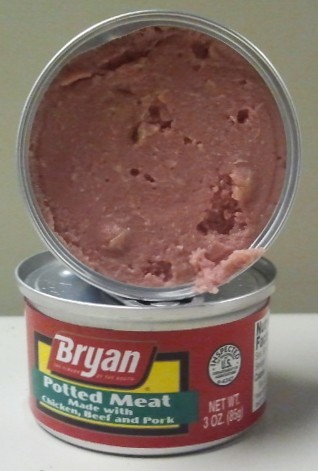In this fuzzy photograph, two tin cans are displayed on a white surface against a green-walled background, possibly a countertop. The can positioned flat on the surface remains unopened, featuring a red label adorned with a green banner that reads "Potted Meat Made with Chicken, Beef, and Pork." The brand name "Bryan" appears prominently in red and white above the green banner. Atop this unopened can sits another can that has been opened, revealing a reddish-colored, unappealing meat mush inside. The label indicates a net weight of three ounces.